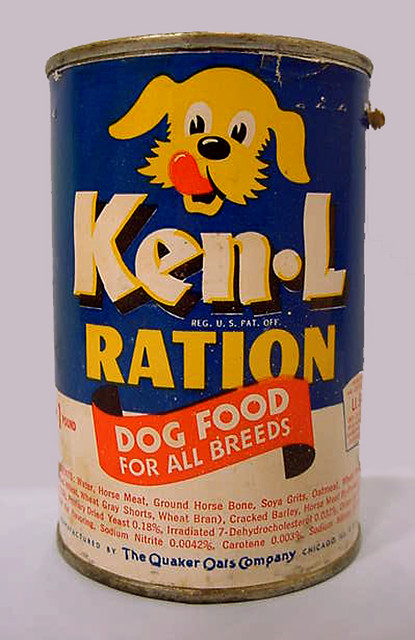This photograph showcases a weathered, antique can of dog food, reflecting its age through its vintage design. The can is prominently adorned with a yellow dog head on the upper portion, set against a blue background. The brand name "Ken.L" is displayed in bold white text with a yellow outline. Beneath this, the word "ration" is featured in yellow text. The lower half of the can transitions to a white background, where a striking red ribbon emblazoned with the text "dog food for all breeds" in white further emphasizes the product's classic appeal. The overall condition of the can, along with the nostalgic design elements, exudes a sense of historical charm.